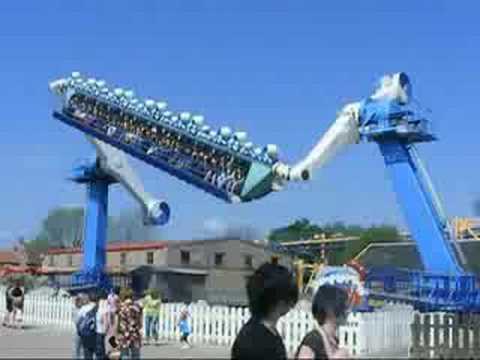The photograph captures a vibrant carnival scene on a clear, sunny day with a flawless light blue sky. Central to the image is a dazzling amusement park ride, featuring two imposing blue arms connected to spinning cranes. These arms support a large, oblong seating area adorned with various blue cylindrical decorations, where numerous people are securely strapped, experiencing the thrilling rotations. The ride operates within a white picket fence, which is surrounded by many onlookers, including two short-haired individuals dressed in black. In the background, a substantial gray building with a red roof is nestled among lush green trees, adding depth to the lively atmosphere. The foreground includes another dark gray fence segment, enhancing the photograph's dynamic composition. The scene is bustling with people, including children, immersing themselves in the carnival's joyous ambiance.